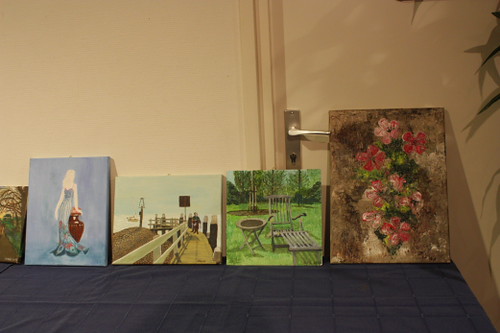The image features five paintings propped up against a beige-colored wall and fire door with a stainless steel, silver lever handle. The artwork is displayed on a table covered with a navy blue tablecloth adorned with square designs, and this setup is partly framed by fronds of a palm-type tree extending from the right side of the image. Each painting varies in size and theme:

1. The partial view of the first, smallest painting includes a brown tree with a green base.
2. The second painting, against a pale blue background, depicts a woman in a turquoise and blue detailed dress, holding what seems to be an urn, her hand resting on her face.
3. The third piece shows a watercolor scene of a boardwalk extending into a bay, with people walking and standing near the water, flanked by a sand mound and a lamp.
4. Next is a painting of an outdoor yard featuring a grass area with a wooden lounge chair, a table, and a mound of dirt.
5. The tallest and last painting presents a dark brown background with roughly rendered pink and red flowers in acrylics.

The detailed artwork and vibrant table setting contrast beautifully against the plain wall and door, providing a captivating display.